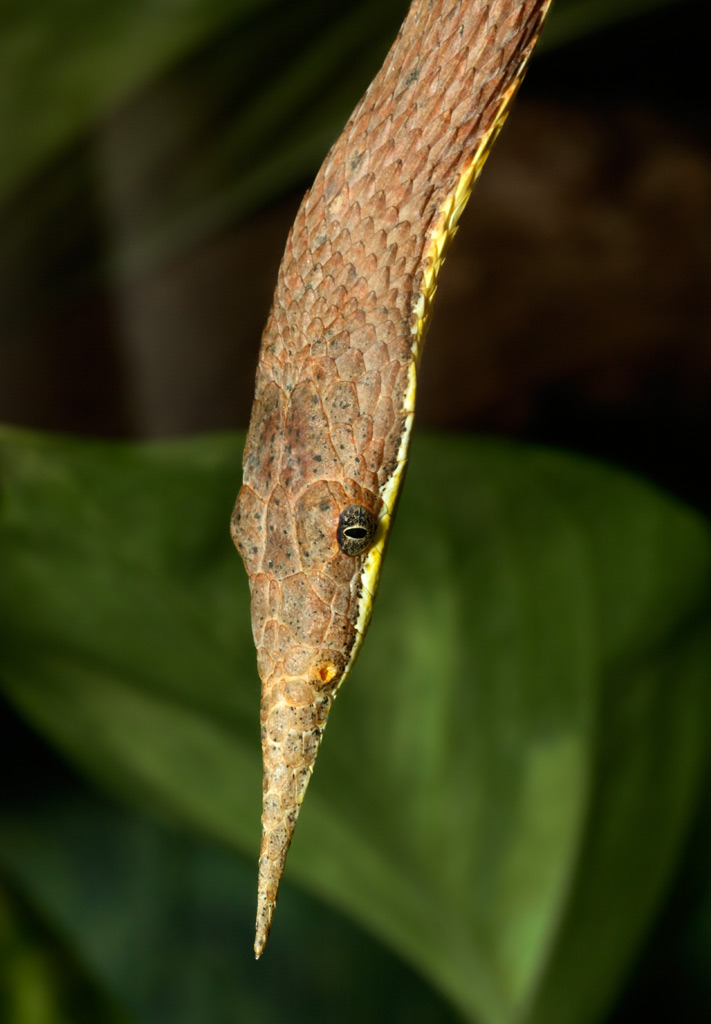This image showcases a close-up of a uniquely altered reptile that resembles a snake. The reptile is dangling vertically from the top center of the frame, positioned against a dark, lush, natural background dominated by large green tropical leaves. Its body features a textured arrangement of brown scales trimmed with green, transitioning to a yellow underbelly. The head of the reptile is particularly striking, with a highly pointed, elongated snout that resembles a downward-pointing spike or unicorn horn, adding an unusual twist to its appearance. This snout, along with its eyes—which appear to be externally set and adorned with a greenish trim around their black, vertically slit pupils—suggests digital alteration. The overall impression is one of natural beauty combined with fantastical elements, creating a captivating and enigmatic scene.